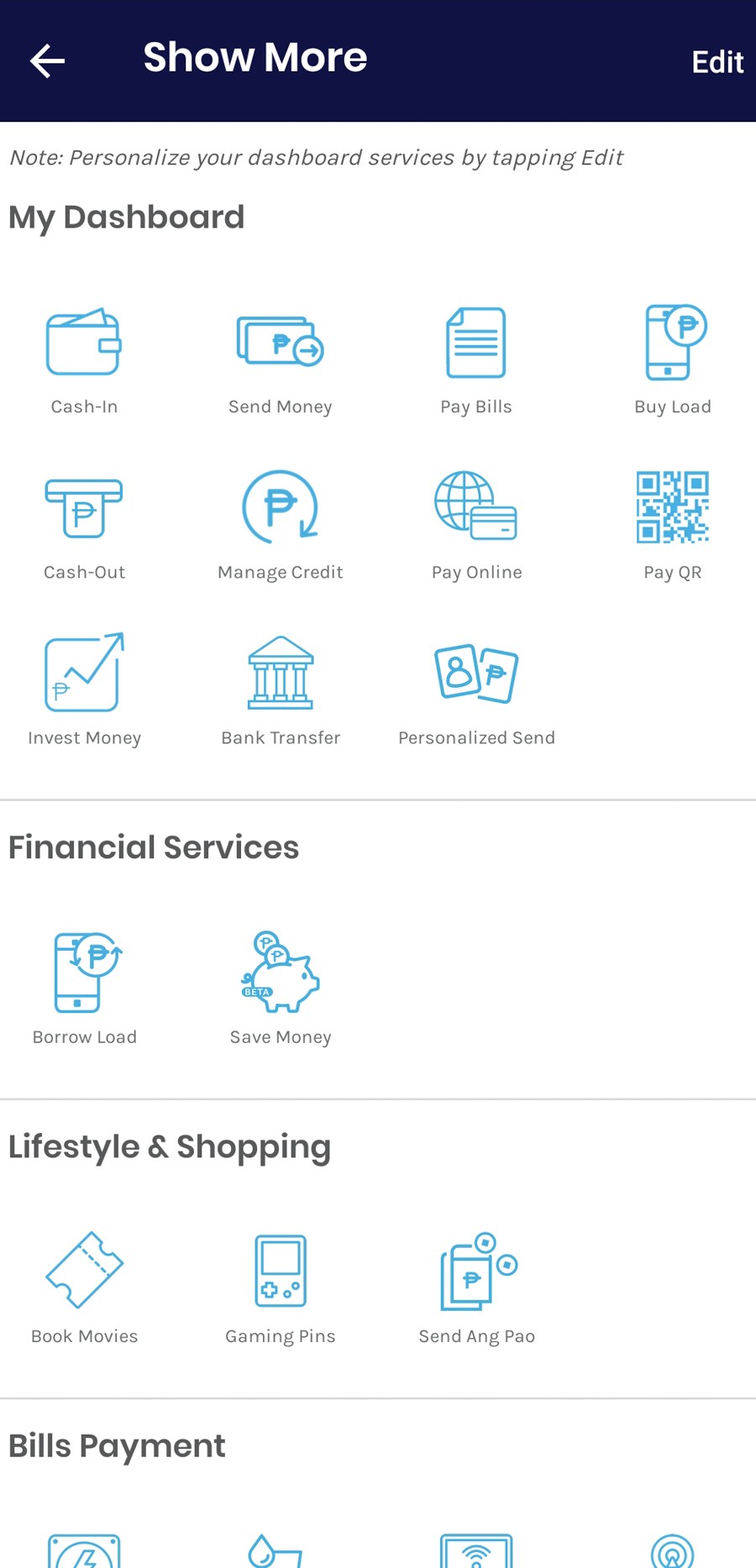The image displays a white background with a detailed view of a personalized digital dashboard interface. At the top left, there's a back arrow, followed by options labeled "Show More" and "Edit." A note instructs users to personalize their dashboard services by tapping "Edit." The main section is titled "My Dashboard" and features several icons representing different actions.

Under "Financial Services," the dashboard includes icons and options such as:
- Cash In
- Spend Money
- Pay Bills
- Buy Load
- Cash Out
- Manage Credit
- Pay Online
- Pay via QR Code
- Invest Money
- Bank Transfer
- Personalize
- Send Money

Additionally, under the "Lifestyle and Shopping" category, users can access:
- Borrow Load
- Save Money
- Book Movies
- Gaming Coupons

A unique feature called "Send AngPayo" (A-N-G capital A, P-A-O with capital P) is also highlighted. Another section is dedicated to "Bills Payment." The overall layout is clean and user-friendly, emphasizing ease of navigation and customization.